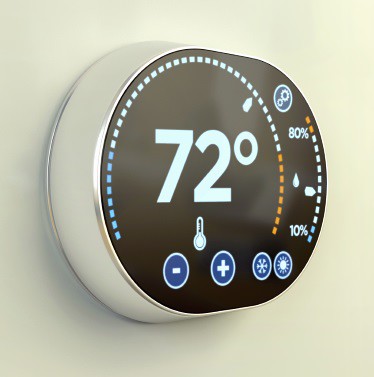This photograph captures a modern thermostat mounted on a pristine white wall, viewed at an angle from the side. The thermostat features a sleek design with white plastic sides accentuated by chrome trim that elegantly frames the device. At its front, it has an oval shape that is flattened on the top, with smoothly rounded left and right sides. The front face of the thermostat is black, providing a striking contrast to its white and chrome elements.

On the left side of the oval face, there is a prominent circular dial that transitions from dark blue to light blue and then to orange. In the center of this dial, large white numbers display the temperature, reading 72 degrees. Directly below these numbers, there is a small thermometer icon, indicating the temperature setting function.

Beneath the thermometer icon are two virtual buttons, each encircled in white but primarily blue, marked with a minus sign on the left button and a plus sign on the right button, suggesting temperature adjustment controls.

To the right of the central dial, another circular meter displays a range from 0% at the bottom to 80% at the top, similarly transitioning in colors from light blue to white to orange. This meter is accompanied by a raindrop icon, indicating its function as a humidity meter.

The overall design and detail of the thermostat suggest a sophisticated and user-friendly device, integrating both temperature and humidity control features in a visually appealing manner.